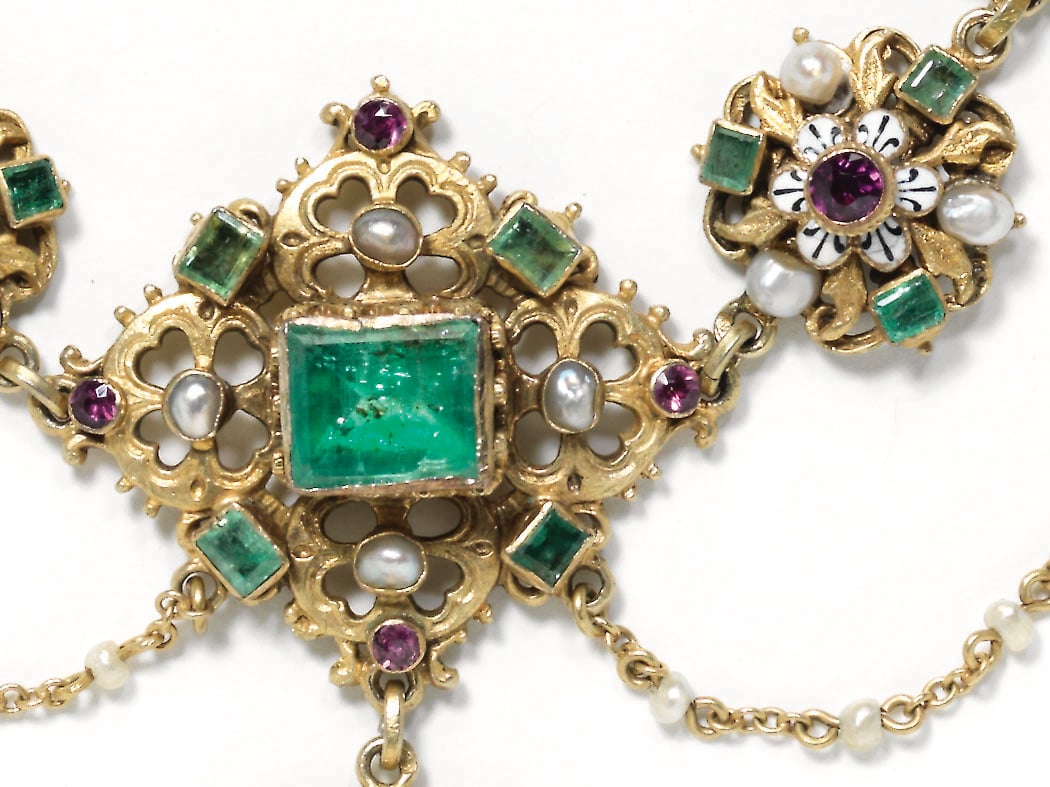The image depicts a detailed and intricate jewelry piece set against a white background. The centerpiece of the jewelry is a diamond-shaped arrangement made of golden metal, designed to resemble interconnected metal flowers. In the core of the diamond-shaped piece lies a large rectangular green gem. Surrounding this central gem are smaller green stones positioned at the points where the metal flowers join. Each metal flower features a white, pearl-like stone at its center, enhancing the floral appearance. At the tips of the diamond shape are circular purple stones, framed by the golden metal.

Chains extend from the central piece in multiple directions: one chain descends from the bottom clasp, another two extend from the lower left and right corners, looping and disappearing out of the image frame. From the upper left and upper right corners, additional chains run off the image. Off to the top right of the main diamond piece, another elaborate section is partially visible. This secondary piece consists of a pink stone encircled by white and golden petals, accented with pearls and green stones. The craftsmanship and complexity of the design hint at a versatile jewelry item, possibly a customizable necklace or brooch, distinguished by its rich palette of green, purple, and white gemstones set in a golden frame.